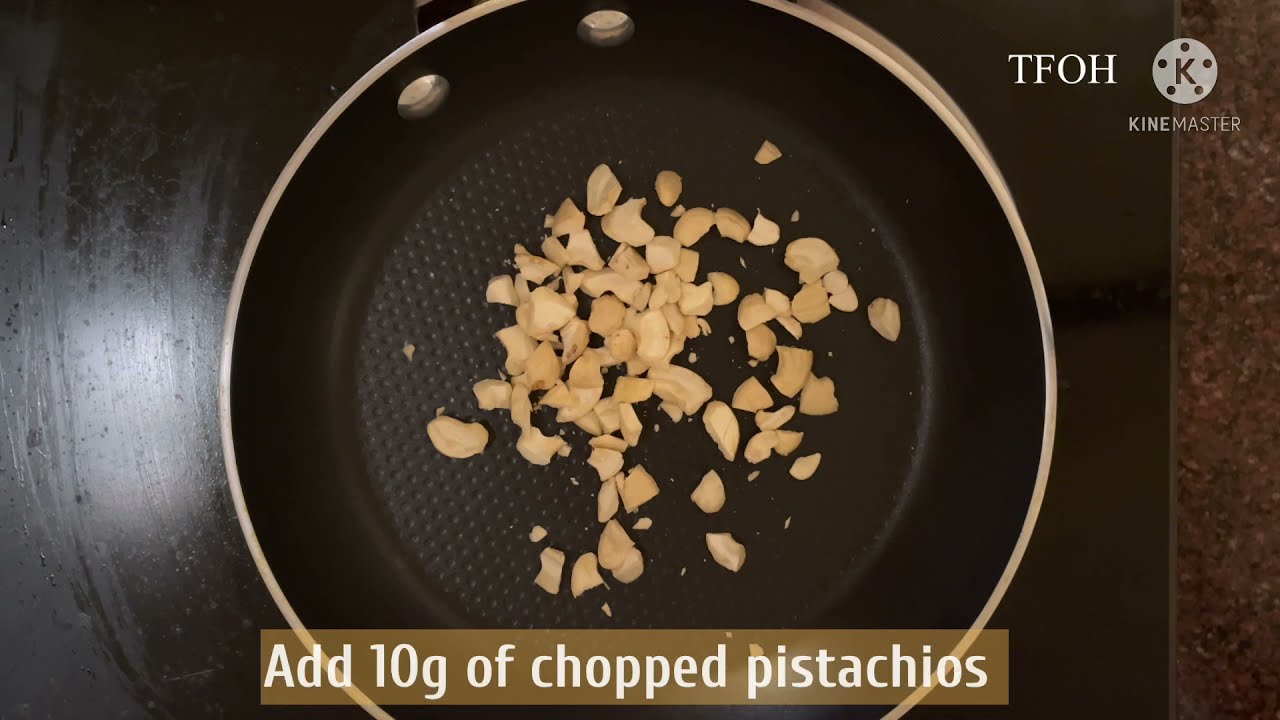This is an overhead view of a frying pan, likely sourced from a cooking video. The pan's interior is black with a non-stick coating and a dimpled pattern at the bottom, while the rims have a goldish hue. Inside the pan, there are crushed or chopped cashews, despite a white caption at the bottom reading "Add 10g of chopped pistachios" in a yellowish or brownish box. The pan is on a black stovetop, partially edged by a marble surface to the right. The handle, equipped with two visible silver rivets, is not in view, giving the pan an almost floating appearance. In the top right corner, the letters "TFOH" are displayed in white capital letters alongside the KineMaster logo, which consists of a circled 'K' with perforations and the word "KineMaster" underneath.